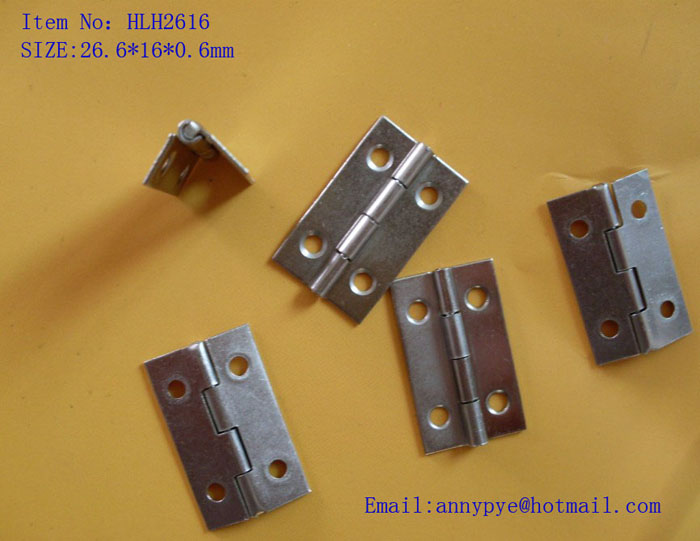This detailed photographic image depicts five small, standard silver-colored hinges arranged on a light brown background. Four of the hinges are laid flat, showcasing both their faces and backs, while the fifth hinge is positioned upright on its pivot. In the top left-hand corner, the text appearing in blue reads "Item Number: HLH2616, Size: 36.6*16*0.6 mm," providing specific product information. Additionally, in the bottom right corner, the email address "annypye@hotmail.com" is displayed in blue, all lowercase. The hinges are presented without any accompanying screws, emphasizing their form and structure against the plain background.